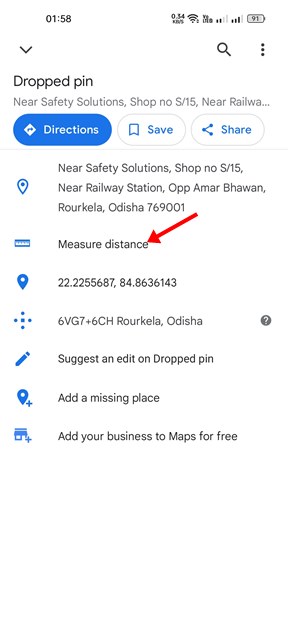A smartphone screen displaying a map search result is captured in this image. The screen is oriented vertically with the status bar at the top showing the time as 1:58 PM, along with phone icons for Wi-Fi, signal reception, and a battery level at 91%. Below the status bar, on the left-hand side, there's a downward-facing arrow, and on the right, icons for a magnifying glass and a vertical ellipsis.

The main content of the screen begins with the bold text "Drop Pin," followed by a gray subtext indicating "Near Safety Solutions Shop, No s/15a, Near Railway," though the text trails off here. Beneath this, three buttons are prominently displayed, labeled "Directions" in blue, "Save," and "Share."

Further down, detailed location information is provided, specifying "Near Safety Solutions Shop, No s/15, Near Railway Station, Opposite AMR Bowon, Rourkela, Odisha, 769001." There is also a feature labeled "Measure Distance," highlighted with a red arrow pointing to it. The coordinates of the pin location are also displayed, followed by options for "Suggest an edit," "Add a missing place," and "Add your business to Maps for free."